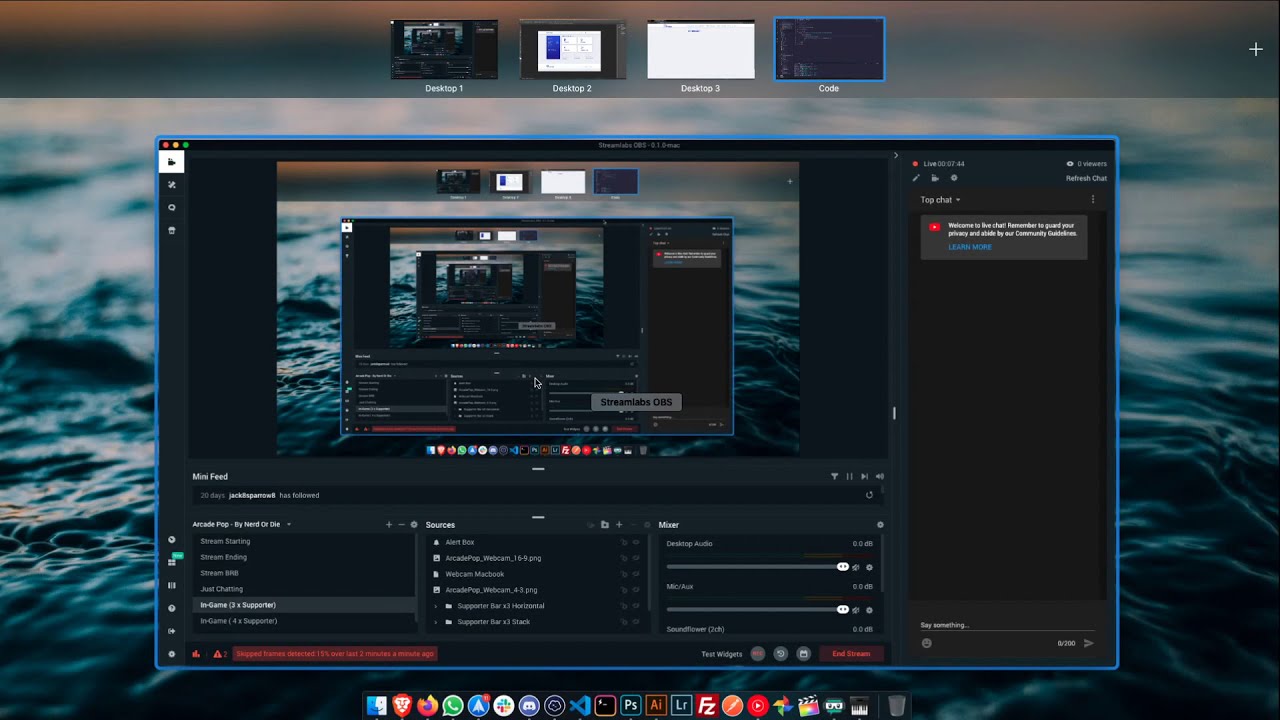This image shows a detailed screenshot of a Mac computer's desktop. The background is a series of dark blue waves, becoming blurrier as they extend upwards. At the bottom of the screen is a centered dock with various application icons, including WhatsApp, Firefox, Discord, and Photoshop. Dominating the center of the screen is a large, dark-colored window. This window displays an endlessly recursive image of the screen itself, creating a "screenshot within a screenshot" effect. This repetition diminishes in size as it seems to recede into the computer. The top part of the screen features a gray bar with multiple virtual desktops labeled "Desktop 1," "Desktop 2," "Desktop 3," and "Code." On the right-hand side of the large window, there is a live YouTube stream bar without any comments. The overall aesthetic is visually complex, with layers of desktop images and a dark, watery background.